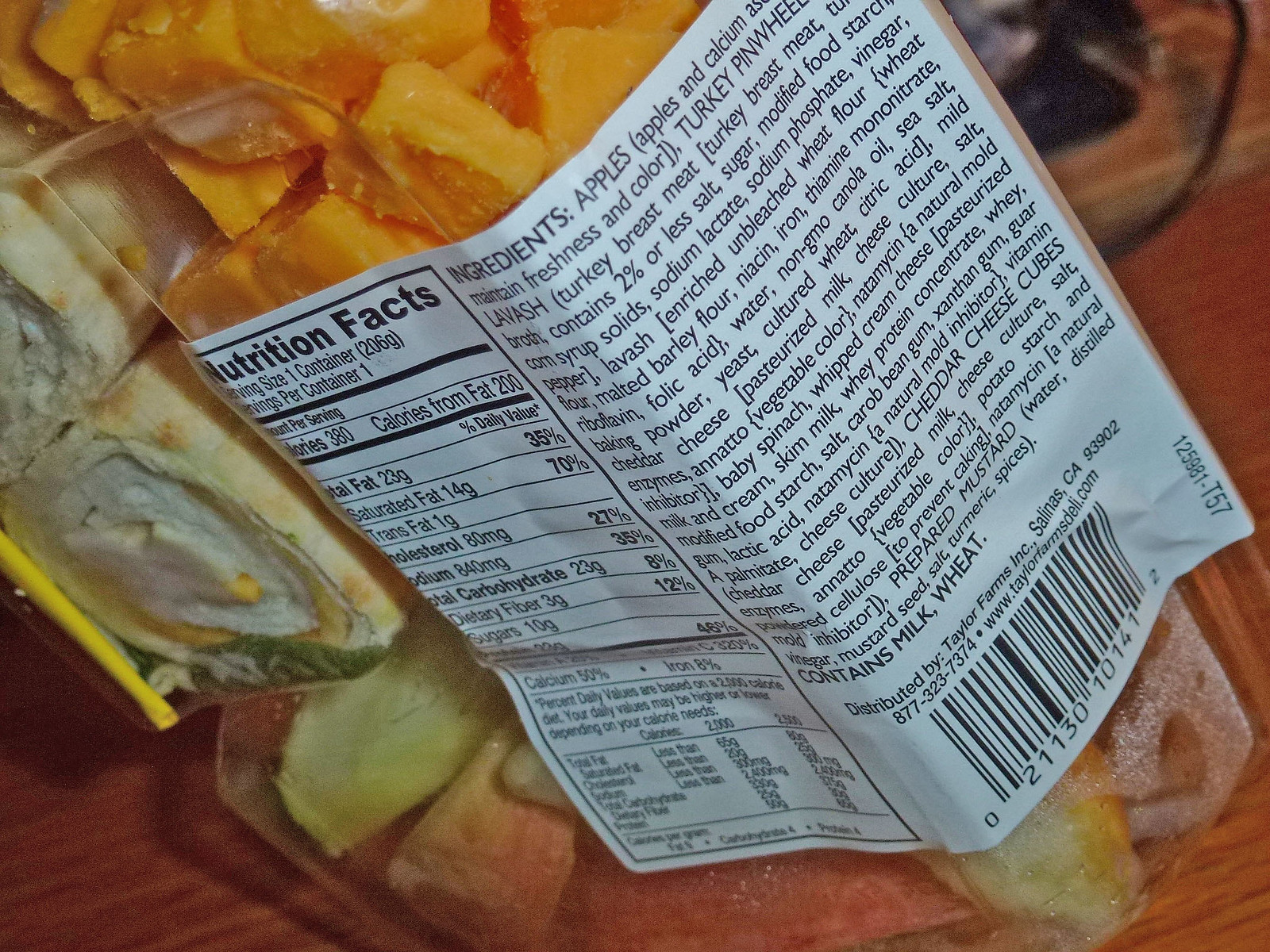This close-up photograph captures the nutrition information on a plastic package of food. Inside the transparent container, you can observe a colorful assortment of food items in hues of orange, beige, and green. Dominating the image is a large white label featuring black text detailing ingredients and nutrition facts. The visible ingredients list includes:

- Apples with calcium to maintain freshness and color,
- Turkey pinwheel with lavash,
- Turkey breast meat (including broth with 2% or less of salt, sugar, modified food starch, corn syrup solids, sodium lactate, sodium phosphate, vinegar, pepper),
- Lavash (enriched unbleached wheat flour, malted barley, niacin, iron, thiamine mononitrate, riboflavin, folic acid, water, non-GMO canola oil, sea salt, baking powder, yeast, cultured wheat, citric acid),
- Mild cheddar cheese (pasteurized milk, cheese culture, salt, enzymes, annatto for color, natamycin as a natural mold inhibitor),
- Baby spinach,
- Whipped cream cheese (pasteurized milk, cream, skim milk, whey protein concentrate, modified food starch, salt, carob bean gum, xanthan gum, guar gum, lactic acid, natamycin as a natural mold inhibitor, vitamin A palmitate, cheese culture),
- Cheddar cheese cubes (cheddar cheese made from pasteurized milk, cheese culture, salt, enzymes, annatto, potato starch, powdered cellulose to prevent caking, natamycin as a natural mold inhibitor),
- Prepared mustard (water, distilled vinegar, mustard seeds, salt, turmeric, spices).

The label also mentions that the product contains milk and wheat. To the left of the label, you can see the nutrition information displayed in black text.